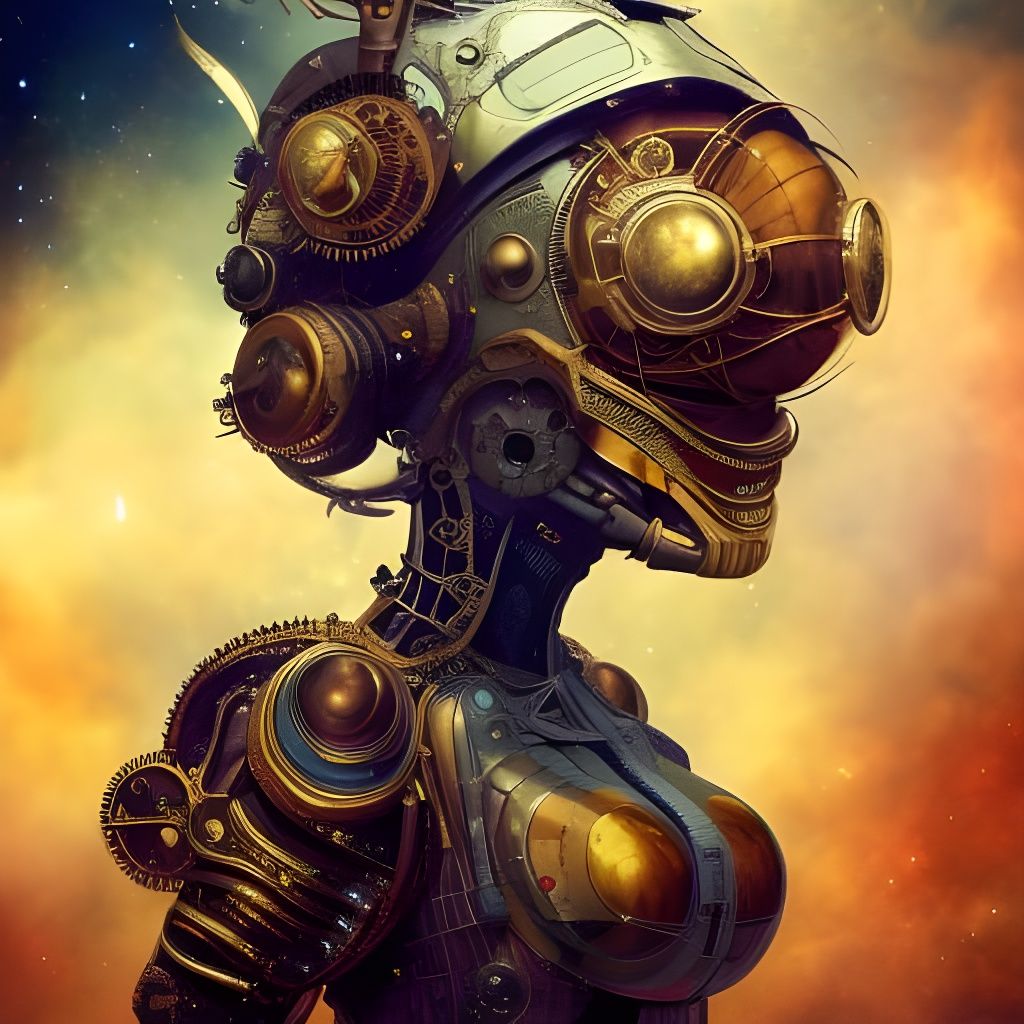The image depicts a very bright and detailed cartoon rendering of a humanoid, female-presenting robot predominantly colored in hues of bronze, brown, and black with reflective gold tinges. The robot is portrayed from just below the bust to the top of the head, though the very top of the head is cut off by the image's frame, which is square in shape and approximately six inches on each side. The robot is facing toward the right, showcasing a side view.

The robot's head features a helmet-like structure with gold dome-shaped caps—in place of ears—and a predominantly gold front, accented by an orange gear on the right side. The eyes are represented by round gold caps, and the nose area is bulbous, almost resembling the shape of glasses. The jawline is depicted in gold with a dark purple and silver underjaw.

The metallic body of the robot is designed with different types of gears, with the bust area highlighted in feminine form using silver material capped with gold at the breasts. The neck appears to be a dark brown, adding to the distinct bronze and black aesthetic. The arms, which are seen extending back behind the robot, also feature large gears.

In the background, the upper left corner shows a small triangle of nighttime sky in blue, speckled with stars. The rest of the sky transitions into various shades of orange, with some spots of white, creating a dramatic contrast that frames the robot and highlights its futuristic design.